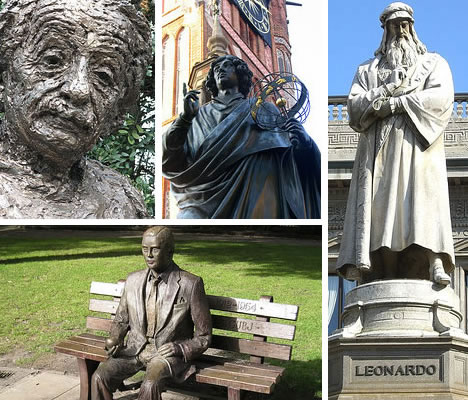The image is a detailed photo collage comprising four distinct photographs of statues, arranged in a square format. In the top left corner, there is a close-up shot of a statue's face, widely recognized as Albert Einstein, exhibiting craggy features and a copperish bronze color, with a mustache and a serious expression making eye contact with the viewer. The top center features an upward-angled view of a dark, almost black statue of a man wearing an ancient Roman-style robe, standing in front of a pink-tinged building. The statue’s right hand is raised with a bent arm, pointing upward, and adorned with long, curly hair. The far right image spans the entire right side of the collage, showcasing a full-bodied, off-white statue identified as Leonardo da Vinci. The statue, perched on a circular pedestal inscribed with "Leonardo," depicts the famed polymath with long hair, a lengthy beard, and a mustache, wearing an older-style hat and a long robe that descends to his ankles. His arms are crossed, with his right hand resting at the bottom of his beard. In the bottom left, a bronze-colored statue of a man in a suit and tie, seated on a park bench, is depicted against a backdrop of green grass and tree shadows. The man gazes forward, with his hands resting on his thighs, one of which appears to be holding a small, indistinct object.